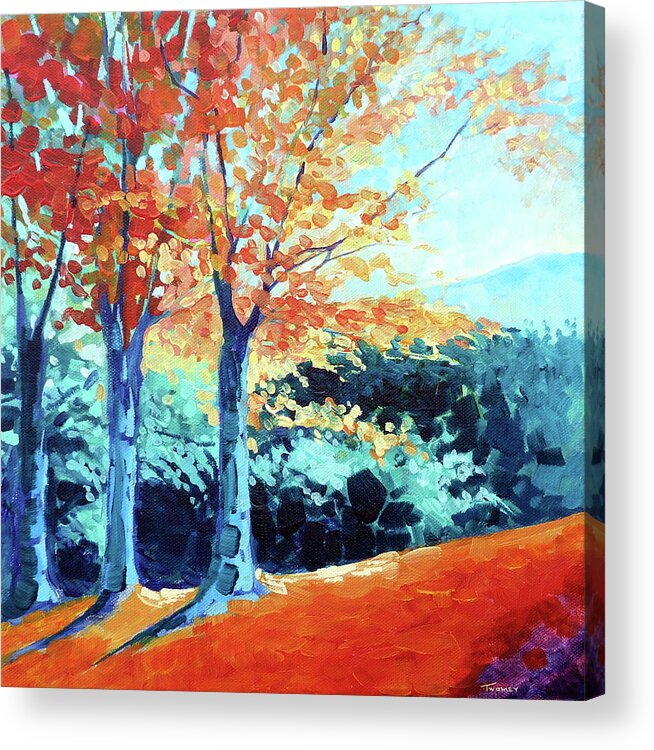This photo features a vibrant and abstract landscape painting displayed on a three-dimensional canvas against a white background. The canvas is slightly angled, revealing its right-hand edge. In the foreground, three blue tree trunks with a canopy of orange, yellow, and red leaves stand prominently on the sloped, orange ground, which extends from the lower right to the upper left. A small purple triangle is noticeable in the bottom right corner of the ground. Behind these trees is a backdrop of abstract, pointillist-style bushes or plants, with colors graduating from dark blue at the bottom to aquamarine in the middle, and returning to dark blue at the top. The background reveals a light blue hill ascending to the right, topped by a clear, blue sky. The painting includes an autograph or signature at the bottom, likely reading "Tomi," "Tumi," or "Twomey" in white, though the exact spelling is ambiguous.